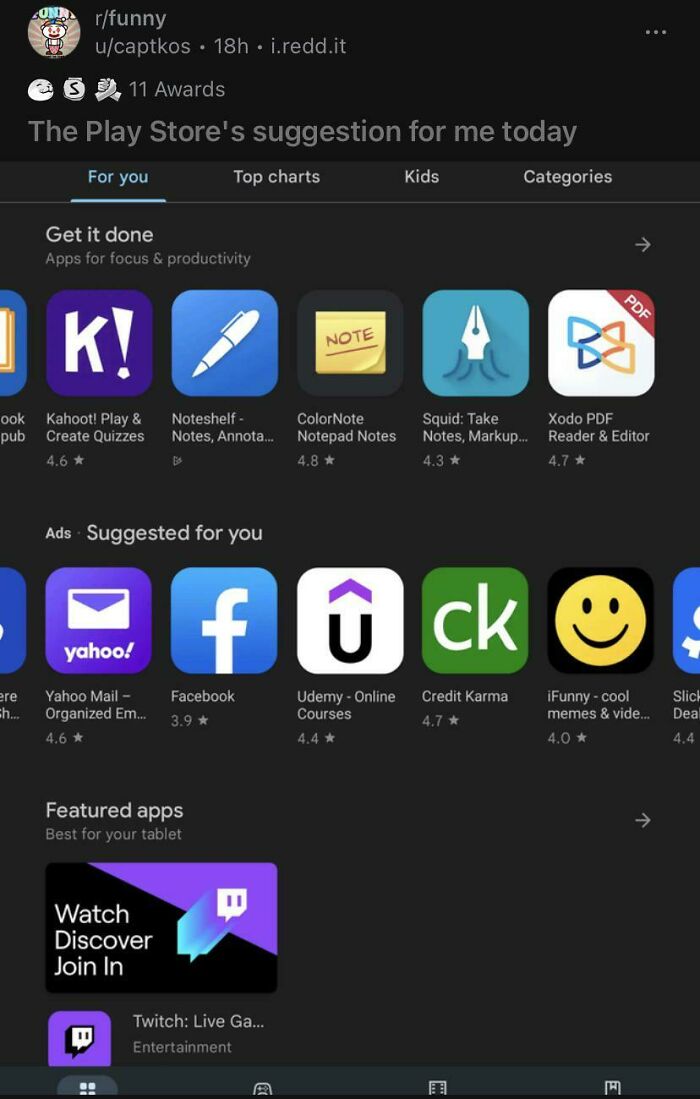Here's a cleaned-up and detailed caption for the given image:

---

This image is a screenshot of the Google Play Store suggestions page, displayed in dark mode. The background is predominantly black with shades of gray used for textual elements.

1. **Top Section**:
   - **Reddit Post Preview**: 
     - **Avatar**: Features the standard Reddit character on a brown background.
     - **Subreddit and User Info**: The post is from the subreddit r/funny, posted by the user u/CapCos. Additional details include "18H" (indicating the post is 18 hours old), separated by white dots from the link "i.red.it" and a row of three horizontal white circles on the far right.
   - **Reddit Symbols**: Below this, there are several Reddit icons:
     - **Smiling Whale**: Likely representing the "Wholesome" award.
     - **Pay Icon (with S)**: Possibly indicating a "Silver" award.
     - **Shaking Hands**: Indicating an "Award" or upvoting.
     - **Awards Count**: Shows there are "11 awards."

2. **Middle Section**:
   - **Play Store Navigation Bar**:
     - **Current Tab**: “For you” selected, highlighted in light blue with an underline.
     - **Additional Tabs**: "Top charts," "Kids," and "Categories," which are not currently selected.
   - **Recommendations Banner**: "Get it done, apps to focus and create productivity."
   
   - **App Recommendations Row**: Features app icons and names:
     - Kahoot Play and Create Quizzes
     - Note Shelf, Notes and Annotations
     - Color Note, Notepad Apps
     - Squid, Take Notes, Markup
     - Xodo, PDF Reader and Editor

3. **Advertising Section**:
   - **Label**: "Ads" with "Suggested for you."
   - **Advertised Apps Row**: Includes 
     - Yahoo Mail, Organized Email
     - Facebook
     - Udemy Online Courses
     - Credit Karma
     - iFunny, Cool Memes and Videos
     - Cut off: Slick Deals
   - **App Ratings**: Each app displayed has its corresponding rating beneath it.

4. **Bottom Section**:
   - **Featured Advertisement**: Promotes “Best for your tablet” apps.
   - **Twitch Ad**:
     - **App Icon**: Twitch logo with text "Twitch Live."
     - **Gradient Background**: A light blue to purple gradient.
     - **Advertisement Text**: "Watch, Discover, Join In."

5. **Footer**:
   - **Mobile Navigation Bar**: Partially visible, indicating the standard Android navigation buttons.